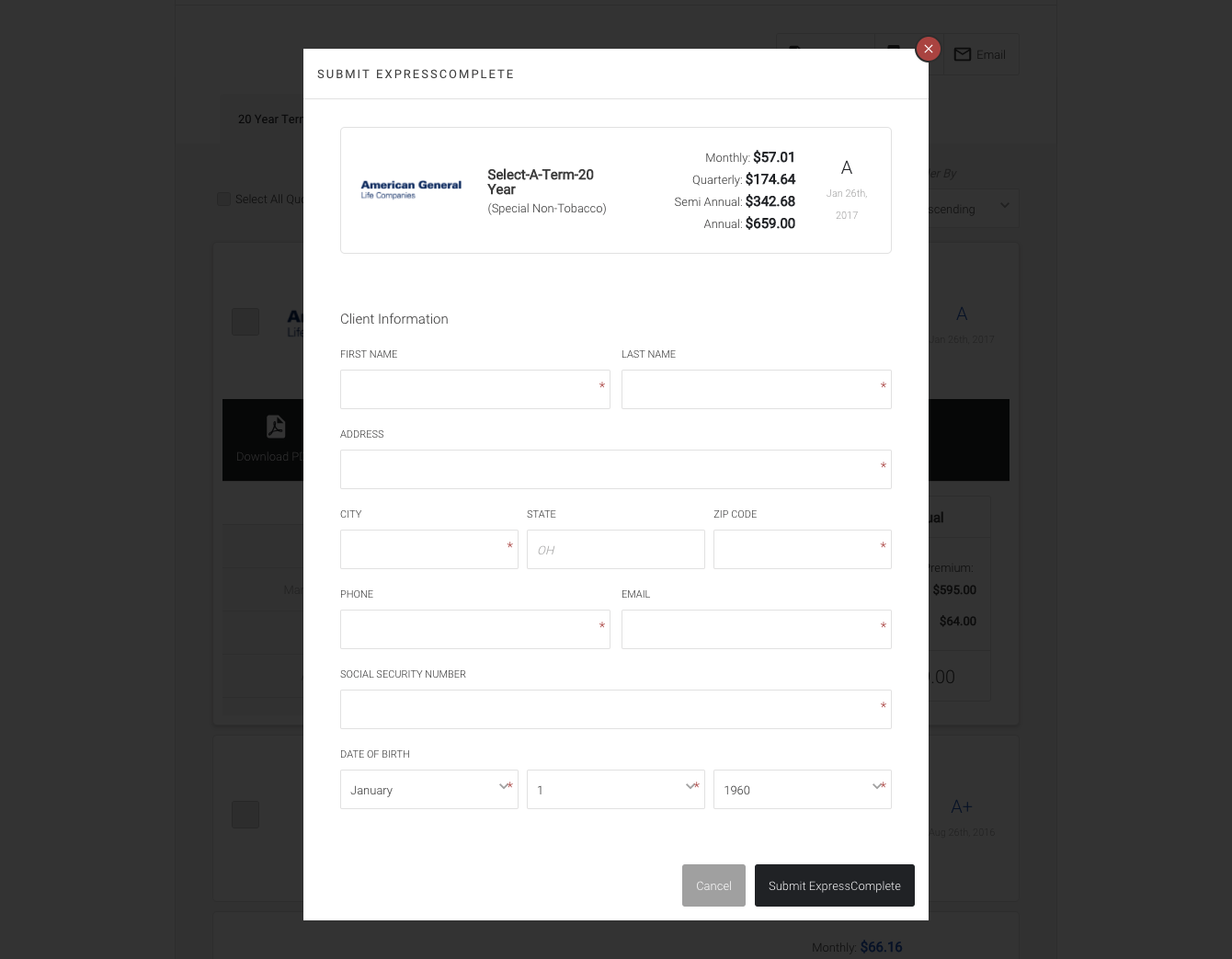A white receipt occupies the majority of the screen, obscuring any underlying content. The background is deliberately darkened to emphasize the receipt, ensuring the background text remains unreadable. At the top-left corner of the receipt, the phrase "Submit Express Complete" is visible in gray text. Below this, there is a box labeled “American General Life Companies” (though the text is slightly unclear). It mentions various insurance term options, specifically "Select a Term, 20 Year, Special Non-Tobacco."

The receipt lists the premium payment possibilities as follows: Monthly - $57.01, Quarterly - $174.64, Semi-Annually - $342.68, and Annually - $659. The date "January 29th, 2017" is noted, possibly indicating the annual renewal date. 

Sections for client information remain blank, including fields for First Name, Last Name, Address, City, State, Zip Code, Phone, Email, Social Security Number, and Date of Birth (with an example date provided as January 1st, 1960). At the bottom of the receipt are options to cancel using a gray button or submit using a black button.